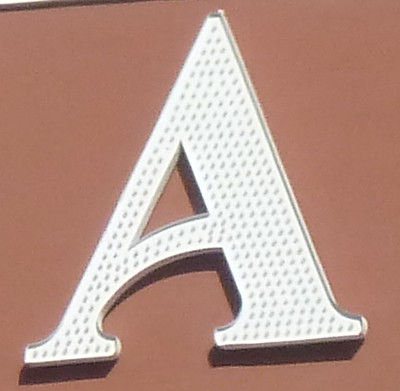The image is a roughly square composition featuring a three-dimensional, stylized letter 'A' set against a dark coral, brownish-reddish background. The letter 'A' appears to be the type of raised letter one might find on a building facade or billboard. It is adorned with circular objects that resemble lights, distributed evenly across its surface. A light source from above casts a shadow extending downward, accentuating the letter's three-dimensional quality. The design of the 'A' is in a serif font; the right vertical bar is noticeably thicker than the left, and the crossbar arches in a graceful curve. The base of the letter features wide, prominent serifs, adding to its bold and distinctive appearance.